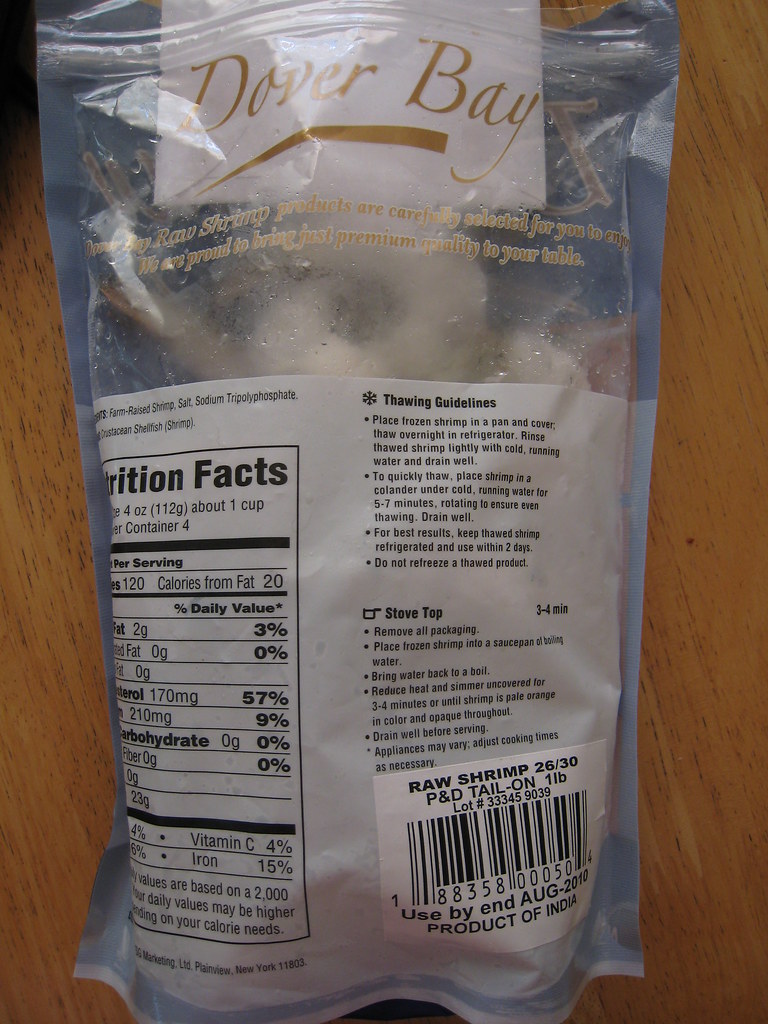This detailed color photograph, taken indoors, showcases a bag of frozen shrimp displayed on a wooden table or countertop. The bag is oriented with the back facing the viewer, revealing a range of information. The upper section of the packaging is clear with gold lettering that reads "Dover Bay," indicating the brand. Below this, a large white panel displays the nutritional facts and ingredients, highlighting that the shrimp are raw and come with preservatives. The panel mentions that the shrimp are a product of India and that the thawing and cooking instructions suggest cooking on the stovetop for three to four minutes. There is also a barcode labeled with the details "26th-30th raw shrimp" and "used by the end of August 2010."